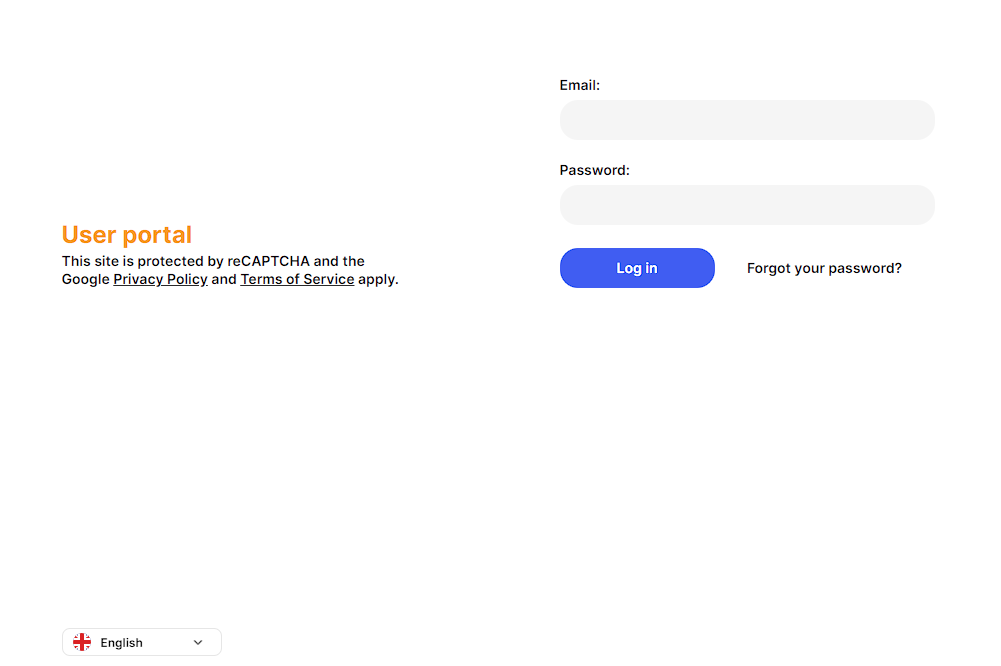Detailed Caption: 

The image features a login page set against a pristine white background. On the left side of the page, there is an orange heading that reads "User Portal" with the word "Users" capitalized. Directly beneath this, there is a statement in black text: "This site is protected by reCAPTCHA." Following this line, the text specifies "Google Privacy Policy" and it is underlined, indicating it is a clickable link. Next to it, also underlined, is "Terms of Service," suggesting another clickable link, followed by the word "apply."

At the bottom left corner of this section, there is a small red "+" icon. Adjacent to the icon, the word "English" is displayed in black, accompanied by a dropdown arrow on the right, enabling the selection of different languages. This entire left-side content is contained within a gray-outlined rectangular box.

On the right side of the page, we see the core login interface. At the top, the word "Email" is written in black above an empty text box. Below this, "Password:" is also displayed in black, followed by another empty text box. These fields are designed to enter the user's credentials.

Beneath the password text box, there is a rectangular blue button with rounded edges, featuring the text "Log In" in white. To the right of this button, in black text, are the words "Forgot your password?" followed by a question mark.

The overall login form appears small in size, which suggests it could be a component of a larger webpage or designed for a tablet interface. The email and password text boxes are empty, with no placeholder or sample text to indicate character limits. Additionally, the left side of the page features the reCAPTCHA security measure, explicitly spelled as "reCAPTCHA" with "re" in lowercase and "CAPTCHA" in uppercase.